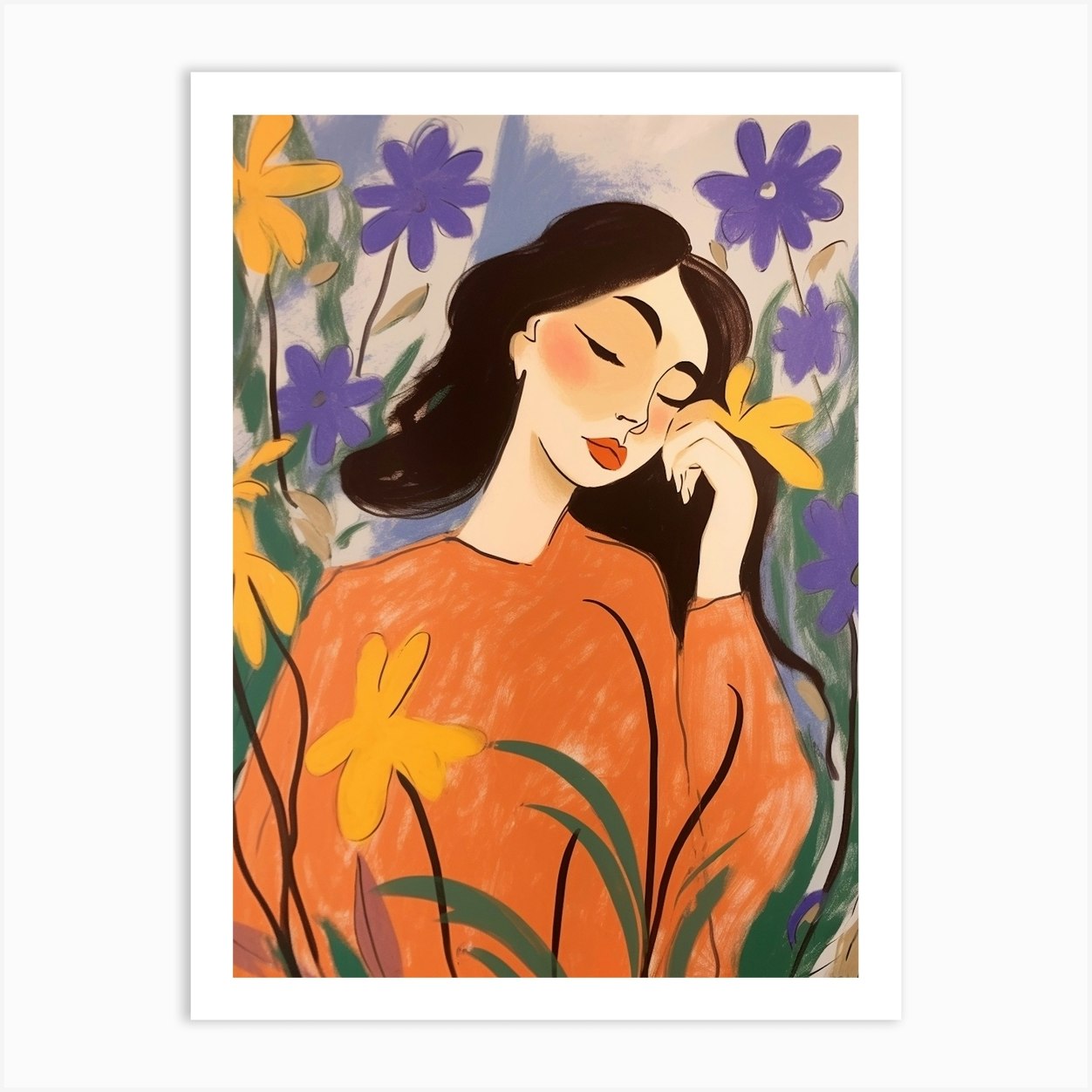This portrait-oriented watercolor painting depicts a serene scene of a woman with long dark hair and vivid makeup, including striking red lipstick. She stands amidst an array of colorful flowers, primarily yellow and purple blooms. The woman, dressed in a long-sleeve orange top, is shown from head to just below the chest. Her right arm is partially visible, while her left arm is raised with her hand delicately resting under her cheek. Her eyes are closed, and she leans slightly to the right, appearing to smell a yellow flower held close to her face. Surrounding her are more yellow and purplish-blue flowers, with stems and green leaves adding to the vibrant, emotional atmosphere of the scene. The painting is framed with a white mat and is displayed against a light gray background on a white wall.